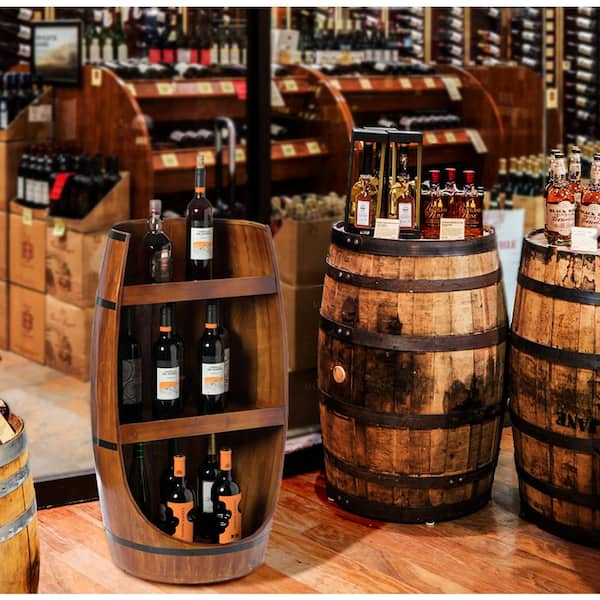In this color photograph, the foreground features three wooden barrels, or casks, with iron fasteners, used for displaying a variety of alcoholic beverages in a liquor store. One of these barrels has been sliced in half to create three wooden shelves, each holding wine bottles. The other two barrels, topped with a mix of liquor bottles and decorative containers, are also prominent. These casks rest on a wooden floor, but the floor in the background appears to be stone tile. Behind the barrels, the store is filled with hundreds of bottles of alcohol, including numerous cases of wine stacked on shelves and in racks, creating a rich tapestry of bottles and boxes that illustrate the store's extensive selection.